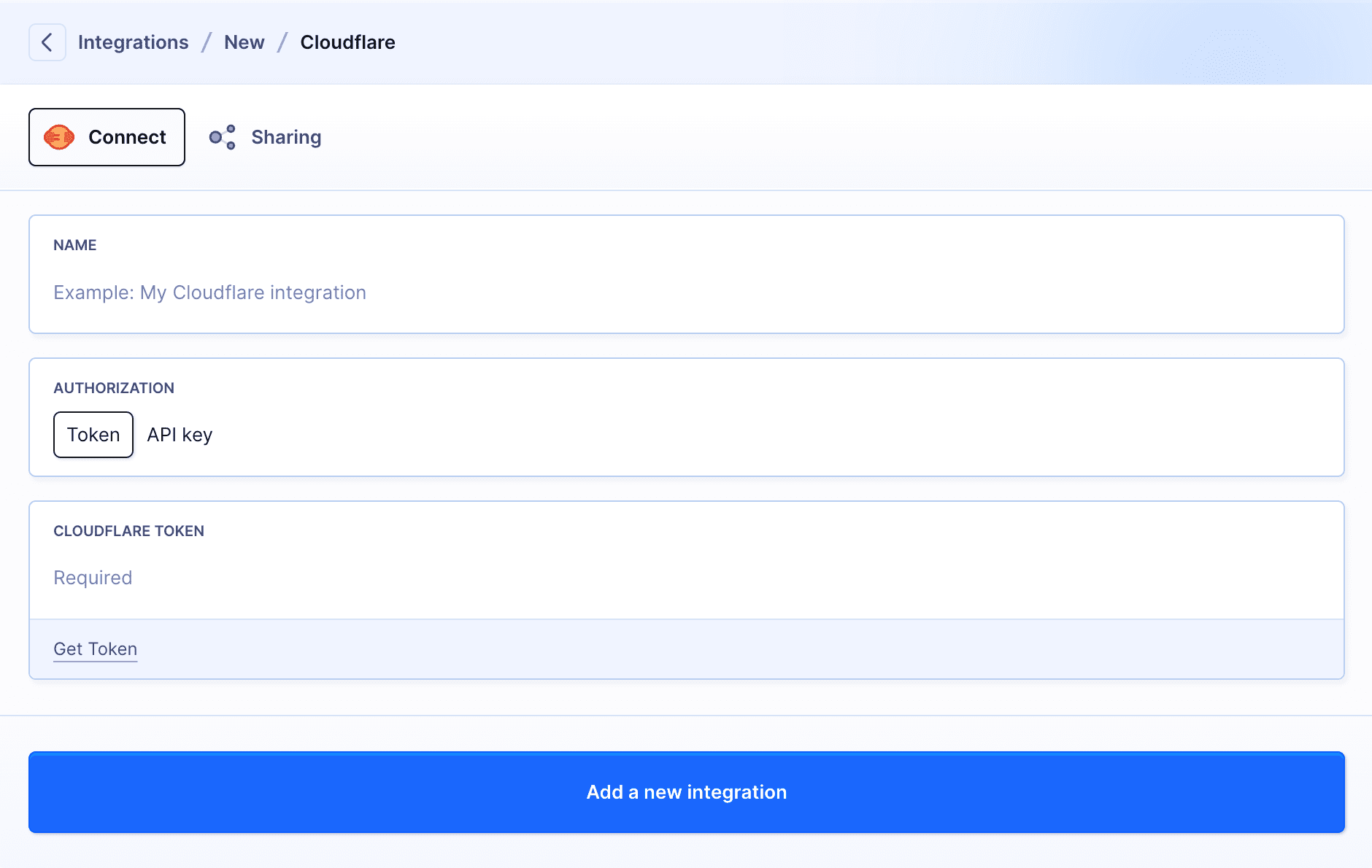The image displays a user interface for a new Cloudflare integration setup. 

At the top is a light blue box labeled "Integration / New / Cloudflare." Directly below this is a section with a box featuring an arrow pointing to the left, and beneath that is another box with a red and orange icon labeled "Connect." 

Adjacent to the "Connect" button is a "Sharing" section highlighted by three interlinked circles, followed by a horizontal line extending across the interface. 

Beneath this line is a text input box labeled "Name," with an example entry "My Cloudflare Integration." Below this is another input box labeled "Authorization," containing a rectangle with the word "Token" in the middle, followed by "API Key." Further down is an additional box stating "Cloudflare Token Required," featuring a light blue highlighted section with "Get Token" written on it. 

At the bottom of the interface, a horizontal light gray line spans the entire width of the image. Below this dividing line is an oversized rectangular blue button that reads "Add a New Integration."